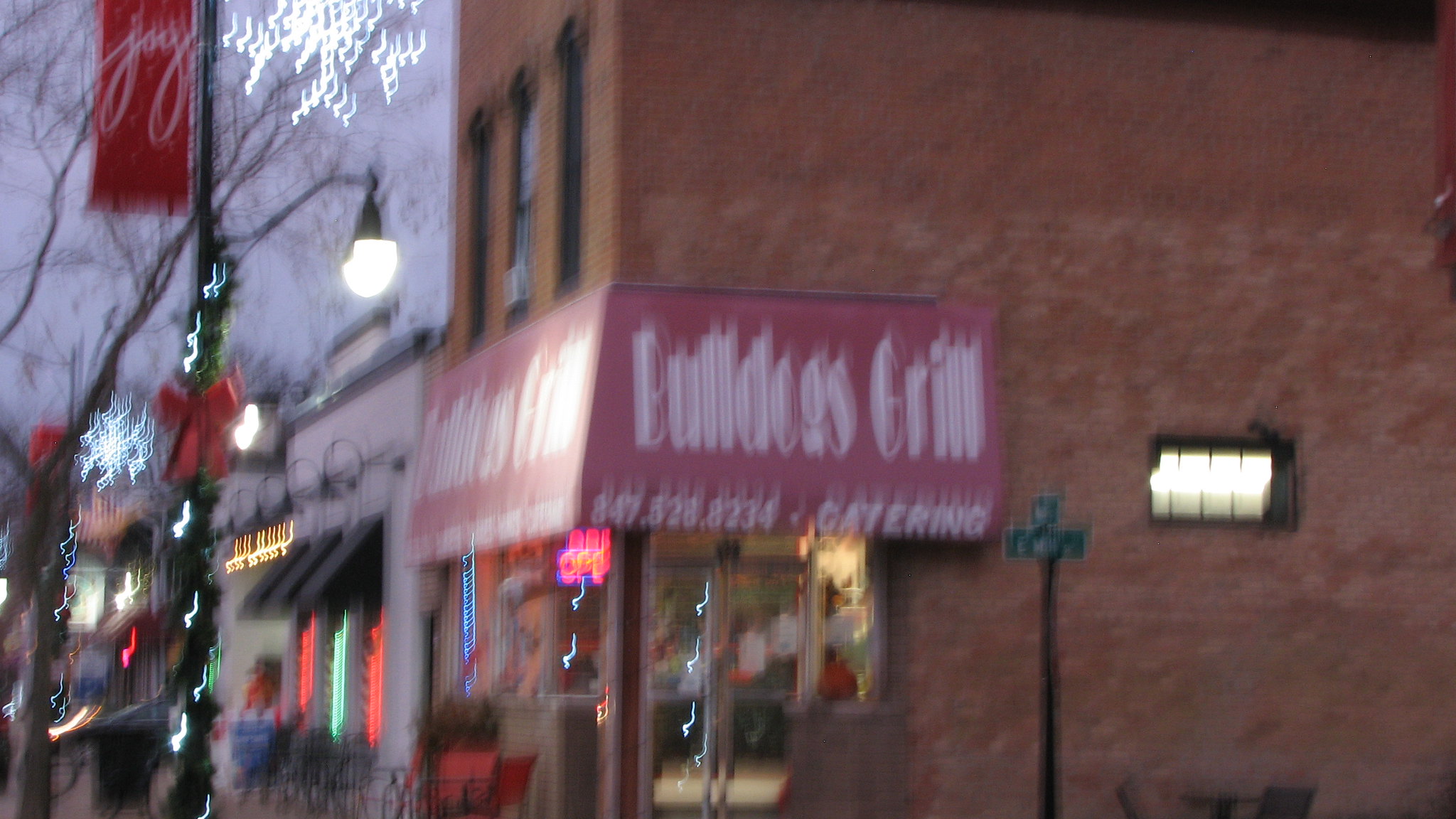This color photograph captures an urban street scene, though it is notably blurred, making specific details challenging to discern. Dominating the right side of the image is a tall building constructed from reddish-grey bricks. At its base, we see a storefront identified by a red sign with white lettering that reads "Lourdes Grill," accompanied by a phone number and the word "catering." Inside the establishment, lights suggest an active restaurant setting. Toward the left side of the frame, a round street light and a tall pole bearing a red sign with additional white writing are visible. Near the bottom of this pole, the indistinct figure of a person can be seen, adding a human element to the scene. Overall, the photograph depicts a bustling streetscape, with its blurred quality evoking a sense of motion and urban energy.